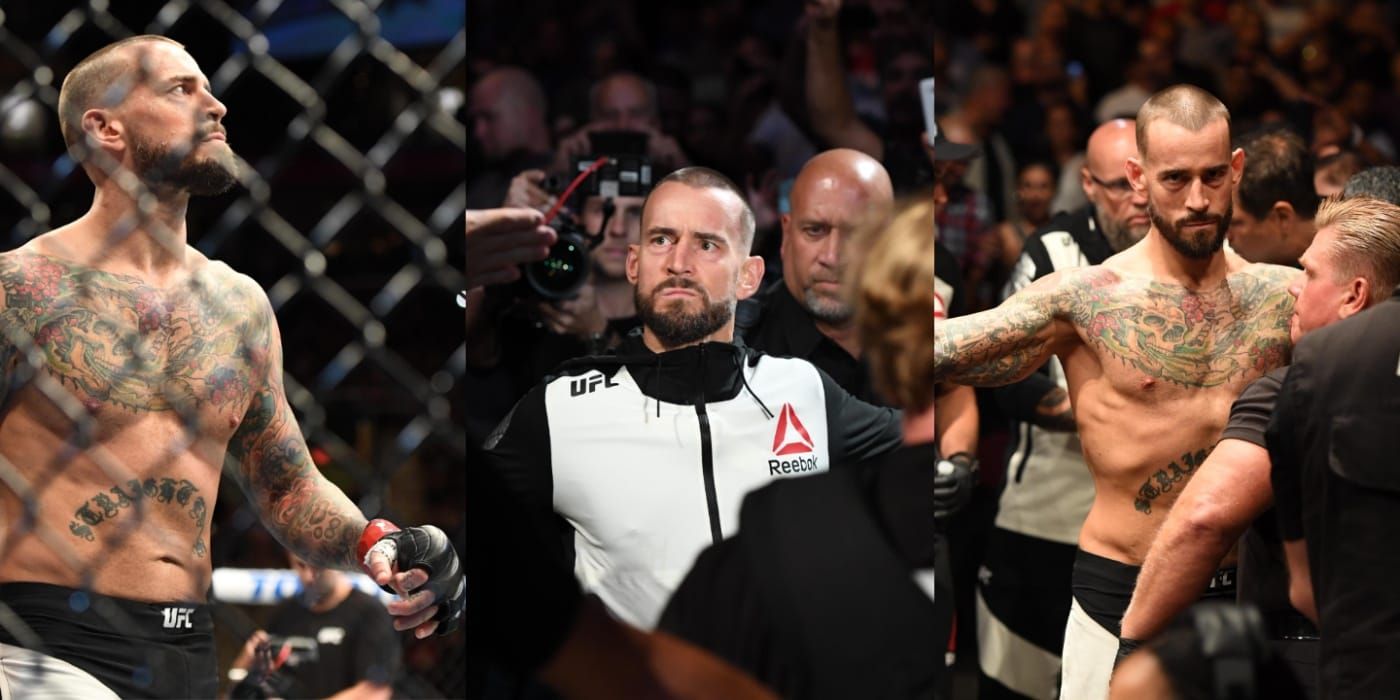The image features a collage of three photographs of the same UFC fighter. In the leftmost picture, the shirtless fighter, distinguished by his tattoos, beard, mustache, and shaved head, stands behind a chain-link fence. In the central photograph, the fighter is in a crowd, wearing a white Reebok jacket with black sleeves and a visible UFC logo on the shoulder. The rightmost picture shows the shirtless fighter again, arms outstretched, displaying his extensive tattoos across his chest and forearms. Behind him is a bald referee with glasses, and in the foreground, there's a man with short, light brown hair and a black t-shirt visible. The images collectively depict moments before an MMA or UFC fight, emphasizing the fighter's readiness and sponsored attire.